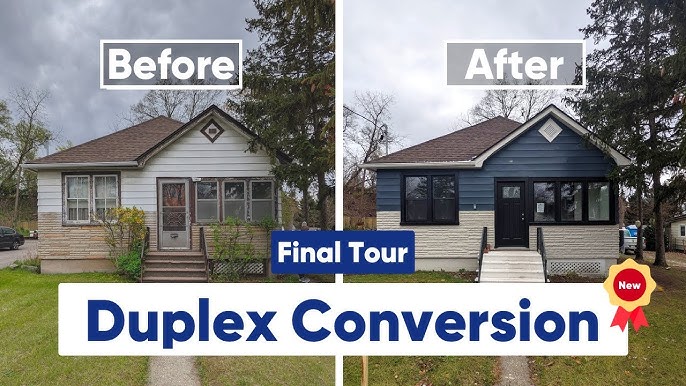This image is a side-by-side comparison showing a house before and after a duplex conversion. At the top of the images, white rectangular boxes labeled "Before" and "After" indicate the transformation stages. The house in the "Before" image features white siding, a beige foundation, a brown shingled roof, a flight of stairs, and a landscaped lawn with trees and plants. The front door is gray, and there are three windows visible on the ground floor.

In the "After" image, notable changes include the upper half of the house being repainted in dark blue-gray, with the lower half and stairs now white. The front door has been replaced with a solid black door, and the trim around the windows has been painted black. Additionally, there is a blue-and-white banner in the center of both images reading "Final Tour" and "Duplex Conversion," accented by a red and yellow ribbon graphic that says "New."

This visually striking transformation highlights the architectural updates and fresh paintwork, giving the house a modernized appearance. The sky is slightly cloudy, and the surrounding trees and lawn remain consistent, although the grass in the "After" image appears in slightly worse condition.